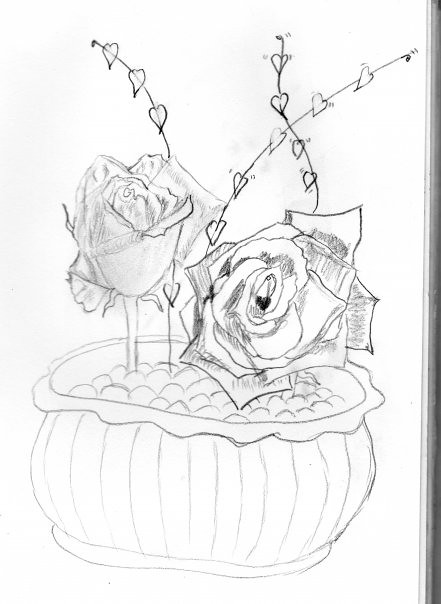This hand-drawn pencil illustration features a detailed depiction of an oblong vase adorned with vertical lines. The vase appears to be partially filled with dirt, represented by wavy, bumpy lines. Two roses emerge from the vase; one stands upright and is partially open, while the other faces forward and is fully bloomed. Within the fully opened rose lies a heart-shaped black object, meticulously shaded with a pencil. Additionally, three vines extend from the vase, each intermittently adorned with small, heart-shaped leaves. Shaded areas, particularly the rose petals, add depth and dimension to the drawing, highlighting the artist's skill and attention to detail.